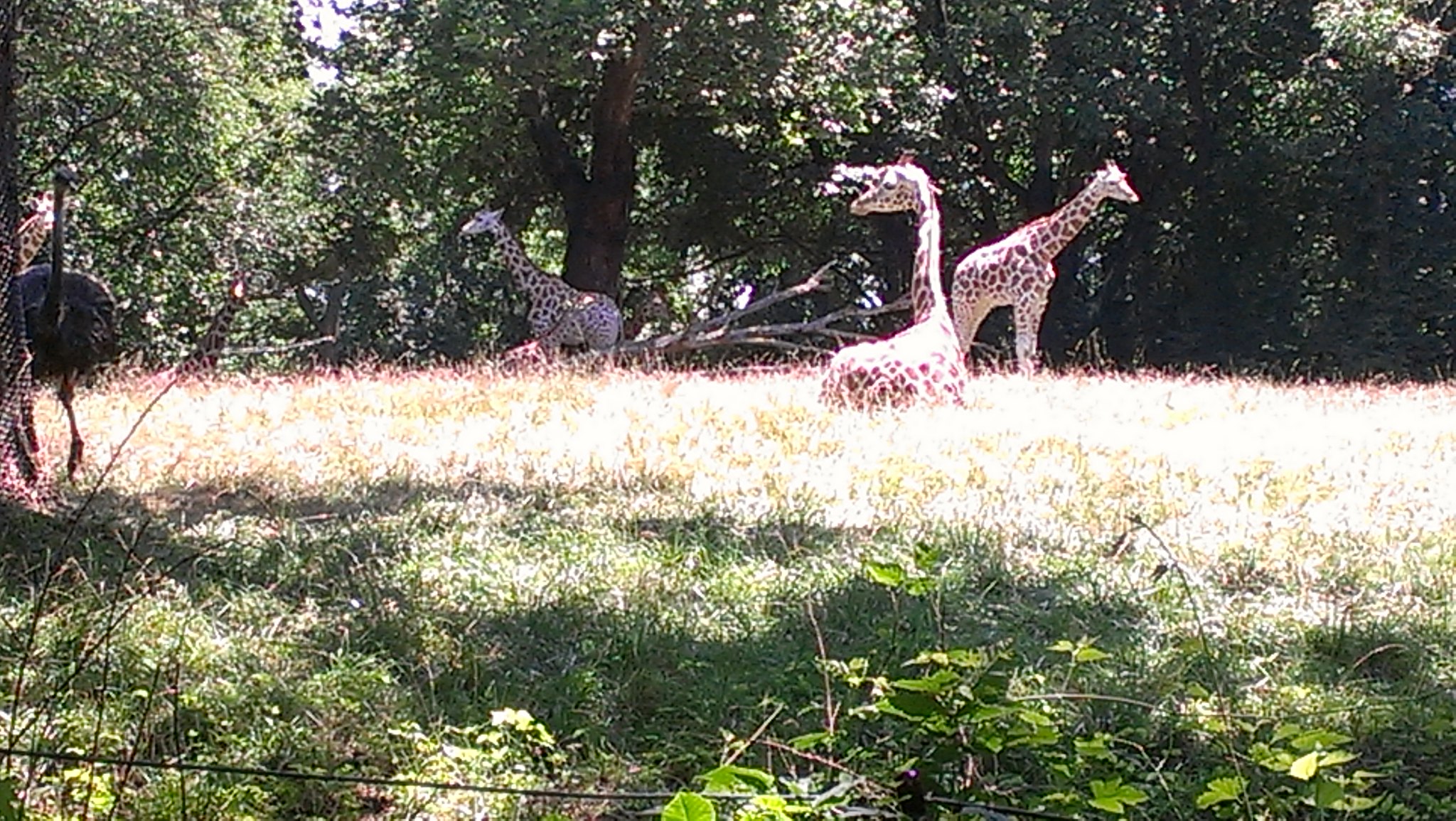The photograph captures a bright, sunny meadow with tall grass and weeds, bordered by a chain-link fence at the bottom. The sunlight illuminates a large portion of the meadow, washing out some areas and casting distinct shadows. Towering trees form a dense, green backdrop, partially shading the field and creating an interplay of light and shadow. In the open meadow, several giraffes are visible, distinguished by their tan and dark brown speckled patterns. One giraffe is sitting down near a tree on the left, blending with the foliage, while two giraffes stand on the right, basking in the bright sunlight. There's also a smaller, fast-moving bird—likely an emu or cassowary—near the left side of the photo, though some descriptions mention an ostrich. In the foreground, a bush with bright green leaves and various plants add texture to the scene. Though some details are washed out by the intense sun, the overall impression is a tranquil, sunlit pasture bordered by rich woodland.